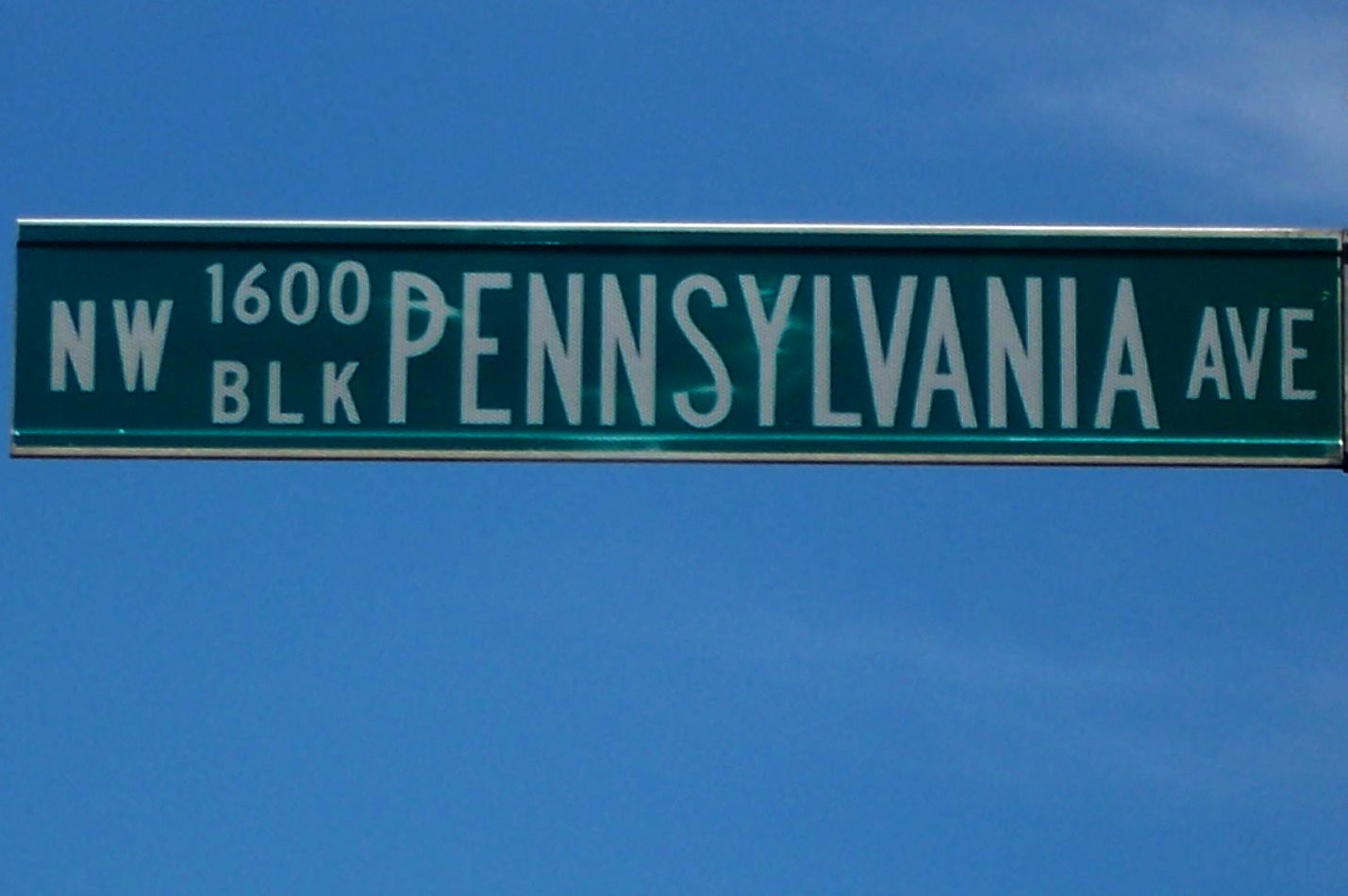This photograph features a traditional green and white street sign commonly seen throughout the United States. The sign displays white lettering that reads "NW 1600 BLK" and "Pennsylvania Avenue." The "NW" indicates the northwest quadrant of the city's grid, and "BLK" is an abbreviation for "block." The background consists of a clear blue sky with a small cluster of white clouds in the upper right corner of the frame. The image is tightly cropped, focusing solely on the street sign, which appears to be made of metal and shows a slight reflection of light on its top and bottom edges. Notably, the photo quality is somewhat blurry and underexposed, with a noticeable bluish tint over the entire image.